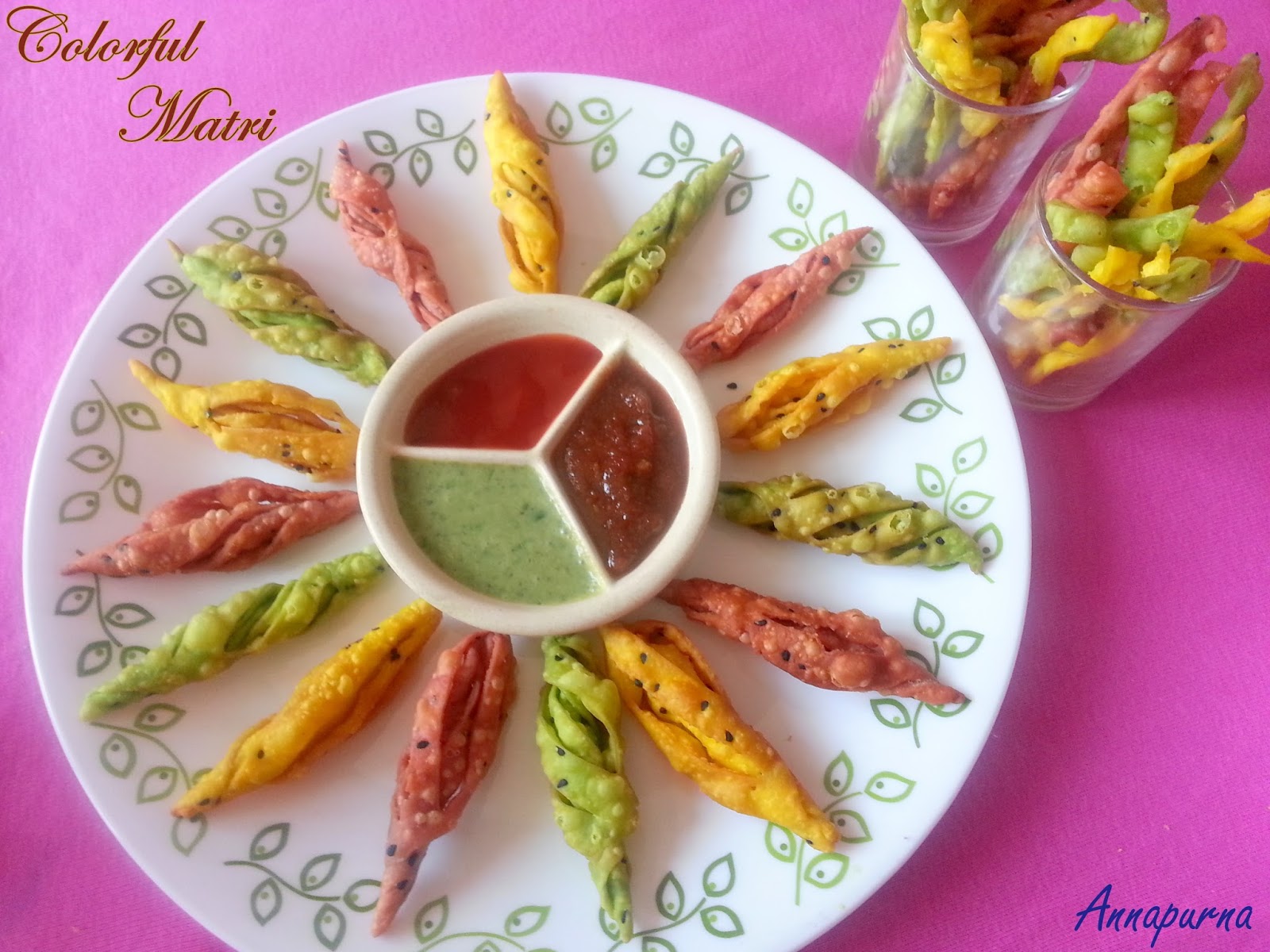The image depicts a vibrant and colorful Indian appetizer platter set against a hot pink tablecloth. The centerpiece is a large white plate adorned with a leafy design around the edges. Arranged in a circular pattern around the plate are twisted fried chips in an array of colors—yellow, green, and pink. These chips, which appear to have seeds or peppers embedded in them, stand vertically, adding a dynamic, wheel-like arrangement to the display. At the center of the plate is a three-compartment dipping bowl. The compartments contain three types of sauces: a bright red sauce, a deep burgundy salsa, and a green sauce. Complementing the spread are two clear plastic cups, located at the top right of the plate, filled with the same multicolored fried chips. The image is framed by text: "Colorful Matri" in red script at the top left corner and "Annapurna" in blue script at the bottom right corner, adding an illustrative touch to the presentation.